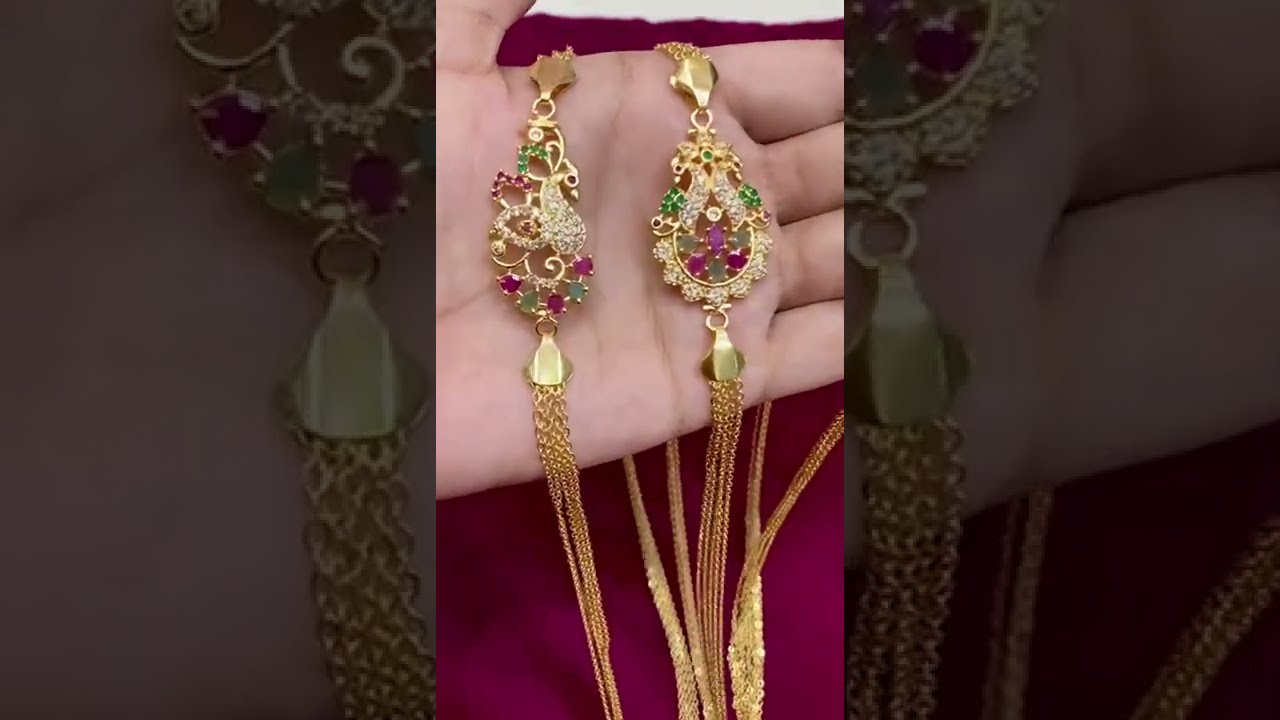The image depicts a close-up of a left hand, fair-skinned and peach-colored, holding two luxurious gold necklaces. The hand is positioned vertically, showing primarily the palm and part of the fingers up to the knuckles, all centered in the frame. Draped over the palm, the two gold necklaces showcase intricate pendants adorned with a variety of jewels. The pendant on the right features a teardrop design with about eight white stones on the bottom half, accented with red and green stones, while the top half is embellished with additional white and green stones. The pendant on the left, in contrast, has a floral design with gold areas resembling leaves interspersed with green and pinkish-purple stones, and small diamond-like crystals. The gold chains, resembling long ropes, are bundled together. The background is a rich magenta cloth, adding depth and highlighting the elegance of the jewelry. The overall effect is a luxurious display of these detailed, jeweled necklaces.